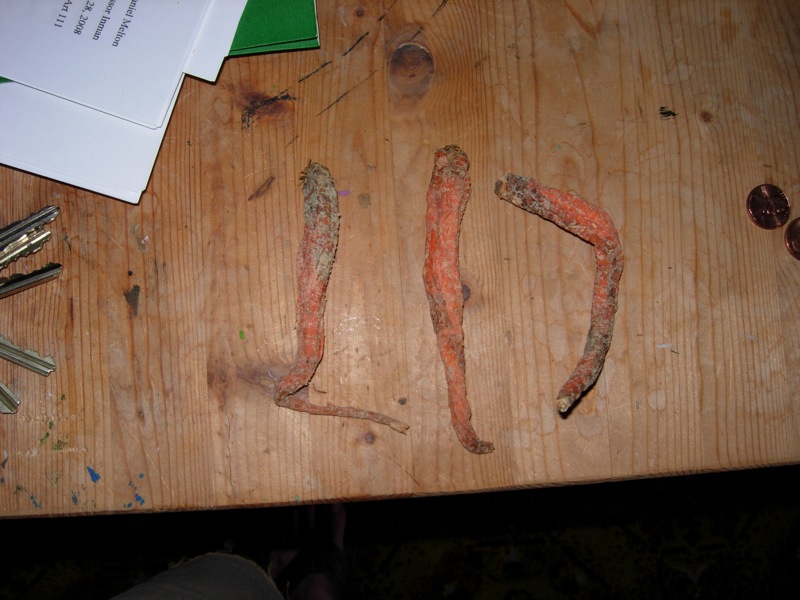A detailed photograph from an overhead perspective showcases three old, shriveled carrots laid out on a worn, light brown wooden table adorned with black marks, stains of ink, and splatters of blue and green paint. The leftmost carrot is heavily misshapen, with a noticeable bend and a greenish-gray hue near the top, indicating mold. The middle carrot is the straightest, though still aged and wrinkled, with some white-green dust covering parts of it. The rightmost carrot exhibits a significant curve and similar moldy discoloration. To the far right of the table, two shiny pennies are visible, one slightly out of focus. At the top left corner, partially covered by a green folder, lie several white sheets of paper with readable text stating "Milton," "Iman," "28, 2008," and "Art 111." The bottom left corner reveals the tips of a set of five keys and a glimpse of the leg of a pair of shorts adding to the cluttered, lived-in appearance of the scene.